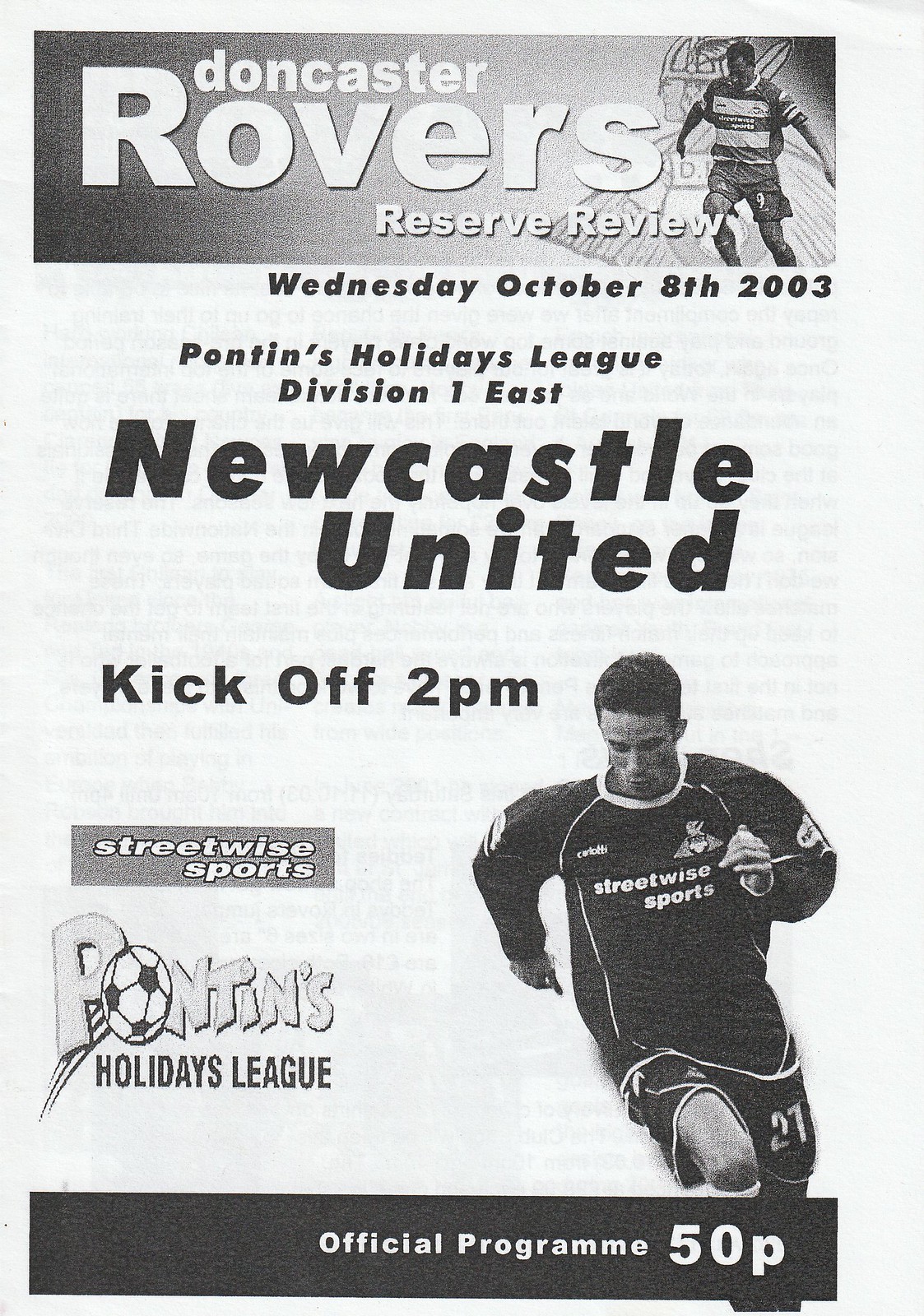Cover of an official program for a soccer game titled "Doncaster Rovers Reserve Review." The top bar features this title along with an emblem resembling a Viking with wings, a sword, and a cape. Below the title, smaller text reads "Wednesday, October 8, 2003" indicating the match details: "Pontins Holiday League Division 1 East, Newcastle United, kickoff, 2 p.m." To the right, a black and white photo of a soccer player is seen. The player is looking down towards the left, with bent knees, wearing a jersey emblazoned with "Streetwise Sports" and black shorts numbered 21. At the bottom left, there are two sponsor logos, one of which is accompanied by a soccer ball icon. The black bar along the bottom states "Official Program 50p."  A section at the back with gray and black background reads "Don Kester, Rovers, Reserve, Resu," next to which lies the player's photograph.